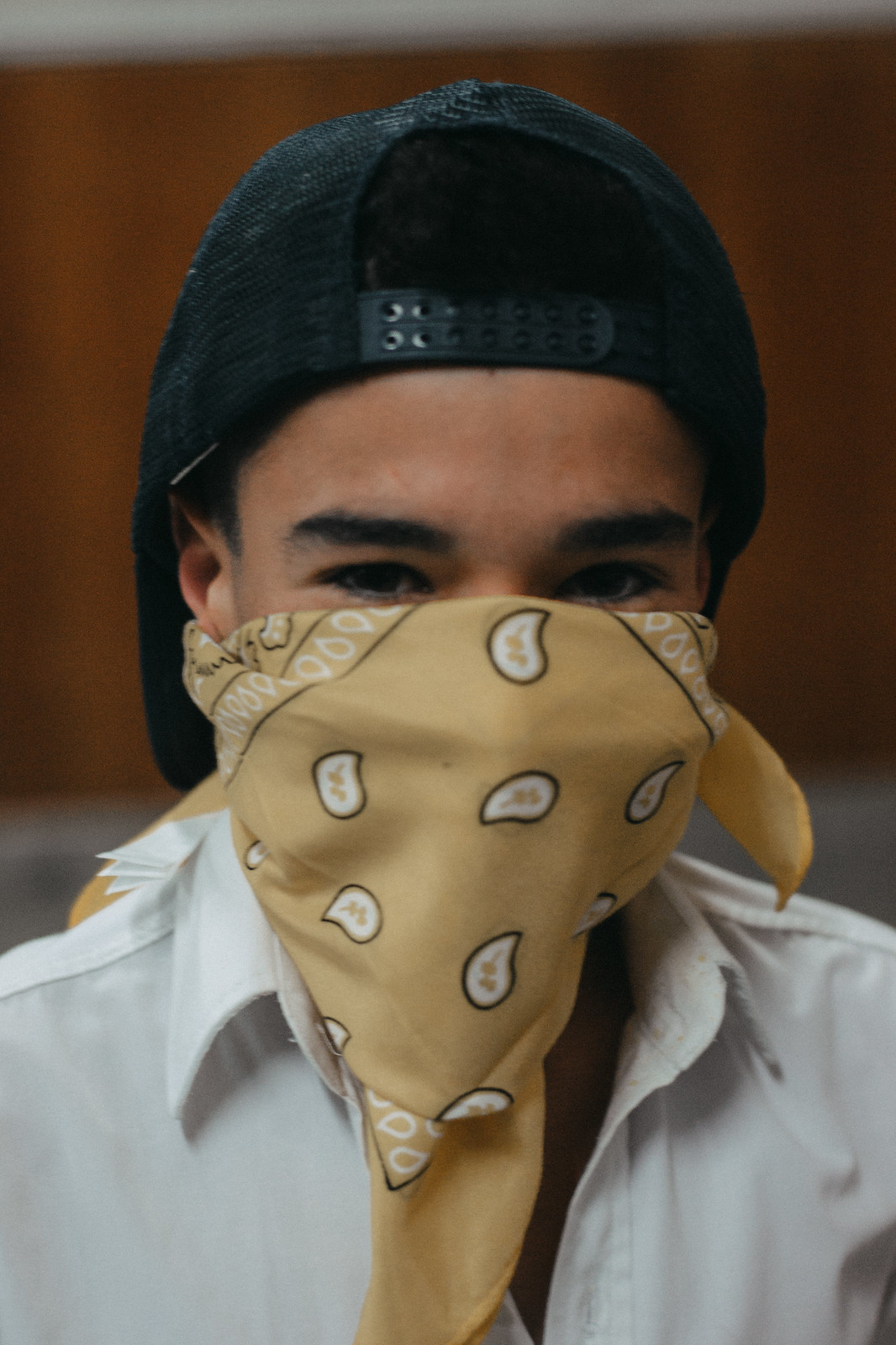The detailed close-up image depicts a tanned-skinned individual of ambiguous gender, concealed partially by a yellow-gold paisley bandana wrapped around the lower portion of their face, covering their nose and mouth. Piercing dark brown eyes and thick, black eyebrows stand out, framed by a backward-worn black baseball cap through which their black hair is visible. The cap, resembling a trucker's hat, features an adjustable strap with a distinctive two-pronged design. The person is dressed in a white, button-down collared shirt, slightly open at the top, against a blurry brown background with a subtle white strip running across the upper portion.